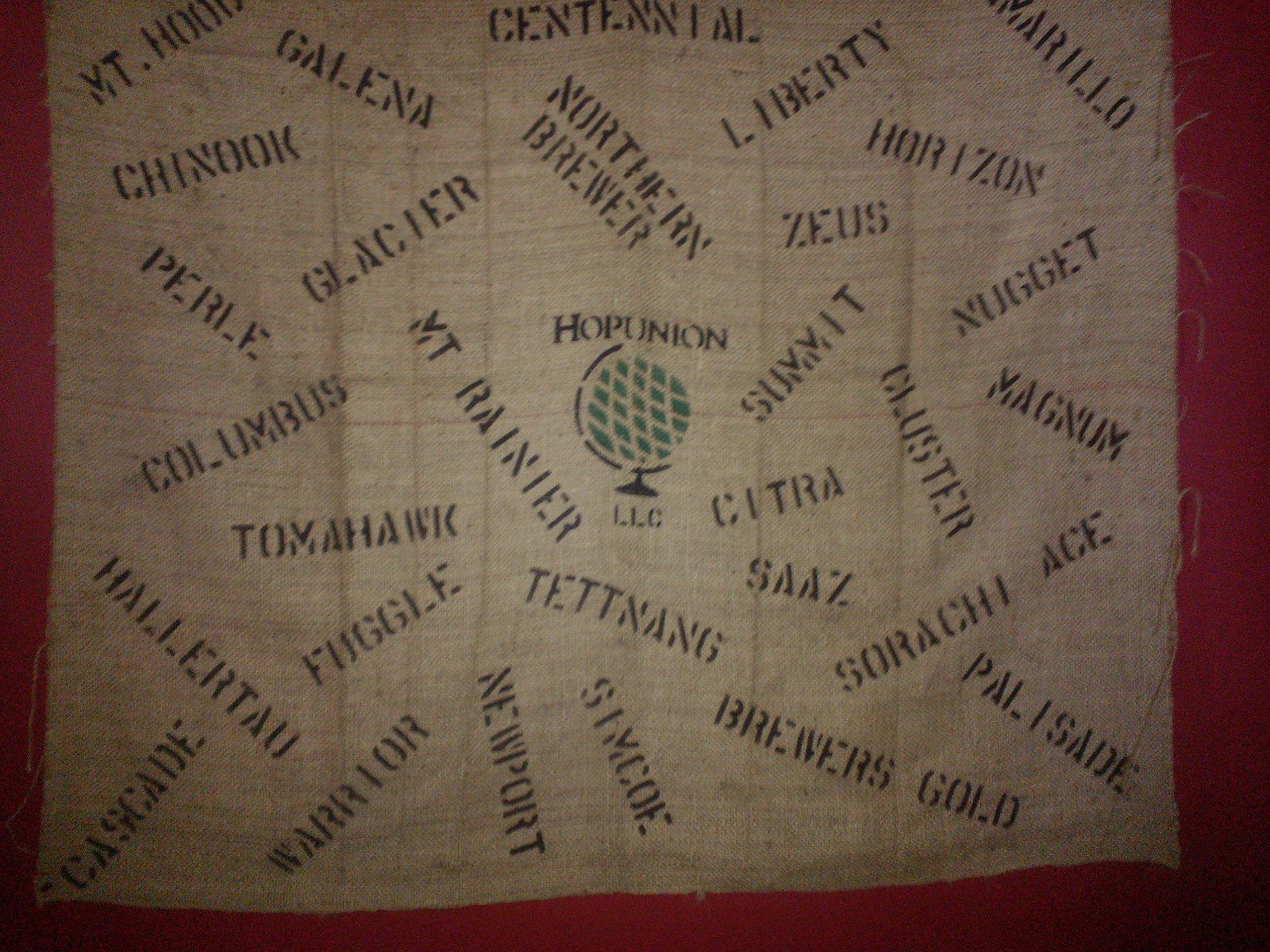Hanging on a solid red wall, the focal point is a rectangular banner made of light gray, somewhat faded canvas. The edges of this textile are noticeably frayed, with loose strings unraveling from the sides. Dominating the center of the banner is a stylized green globe perched on a black stand, above which reads "Hope Union LLC" in black stenciled font. Scattered seemingly at random around the globe are numerous black stenciled names, such as Chinook, Galena, Glacier, Pearl, Columbus, Tomahawk, Fuggle, Citra, Mount Rainier, Saz, Newport, Simcoe, Brewer's Gold, Palisade, Srirachi Ace, Horizon, Zeus, Summit, Nugget, and more. The various names create a visually chaotic yet intriguing display, emphasizing their presence against the backdrop of the solid red wall and the muted, worn material of the banner.